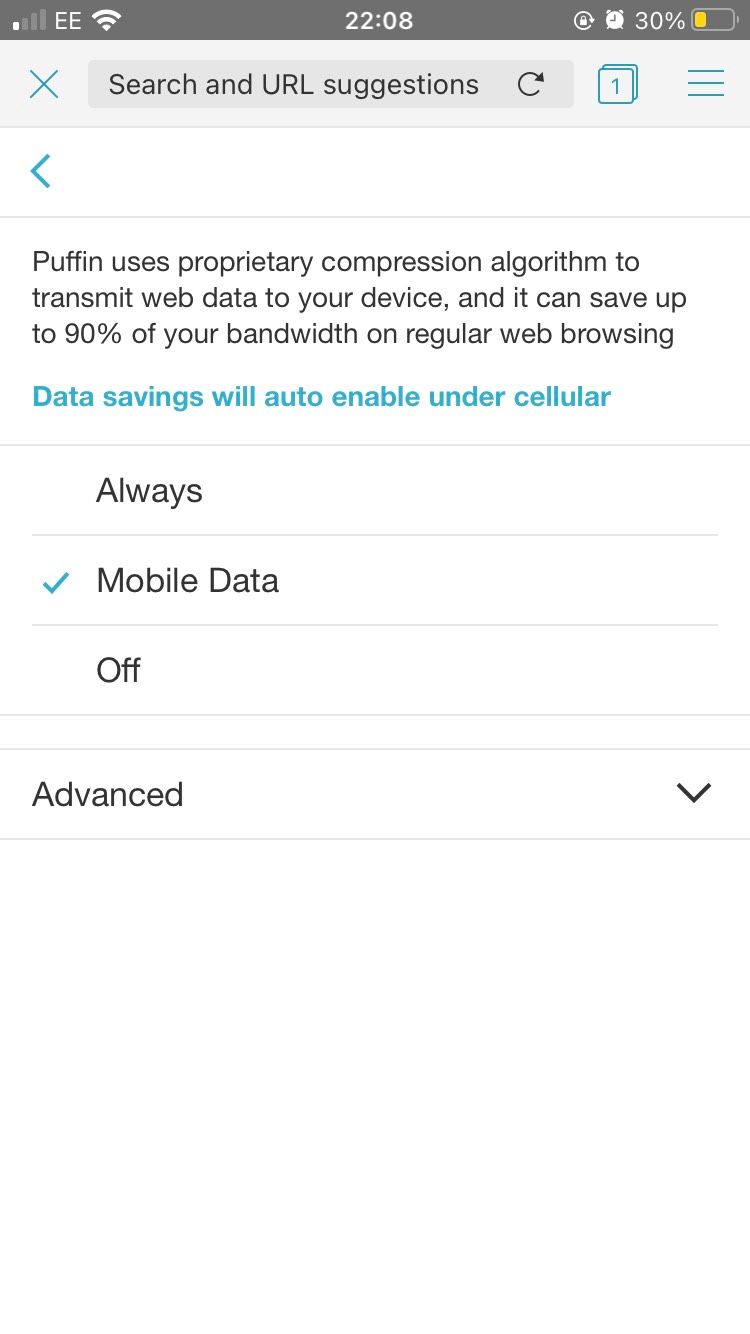The image depicts a search page on an Apple smartphone. At the top, the URL field displays the words "Search and URL suggestions." Directly below this, on the left side, there is a button that appears black but is actually blue. Below the button, black text states: "Parfyn uses a proprietary compression algorithm to transmit web data to your device and it can save up to 90% of your bandwidth on regular web browsing." The background of the image is entirely white. Beneath this text, in a blue or light blue font, is the message: "Data savings will also enable under cellular." Following this, three options are listed: "Always," "Mobile Data," and "Off." The "Mobile Data" option is selected, indicated by a light blue checkmark to its left. At the bottom of the image, there is a dropdown menu labeled "Advanced." Most of the text in the image is written in black, with the exception of the blue text indicating data savings under cellular and the selected option for mobile data.